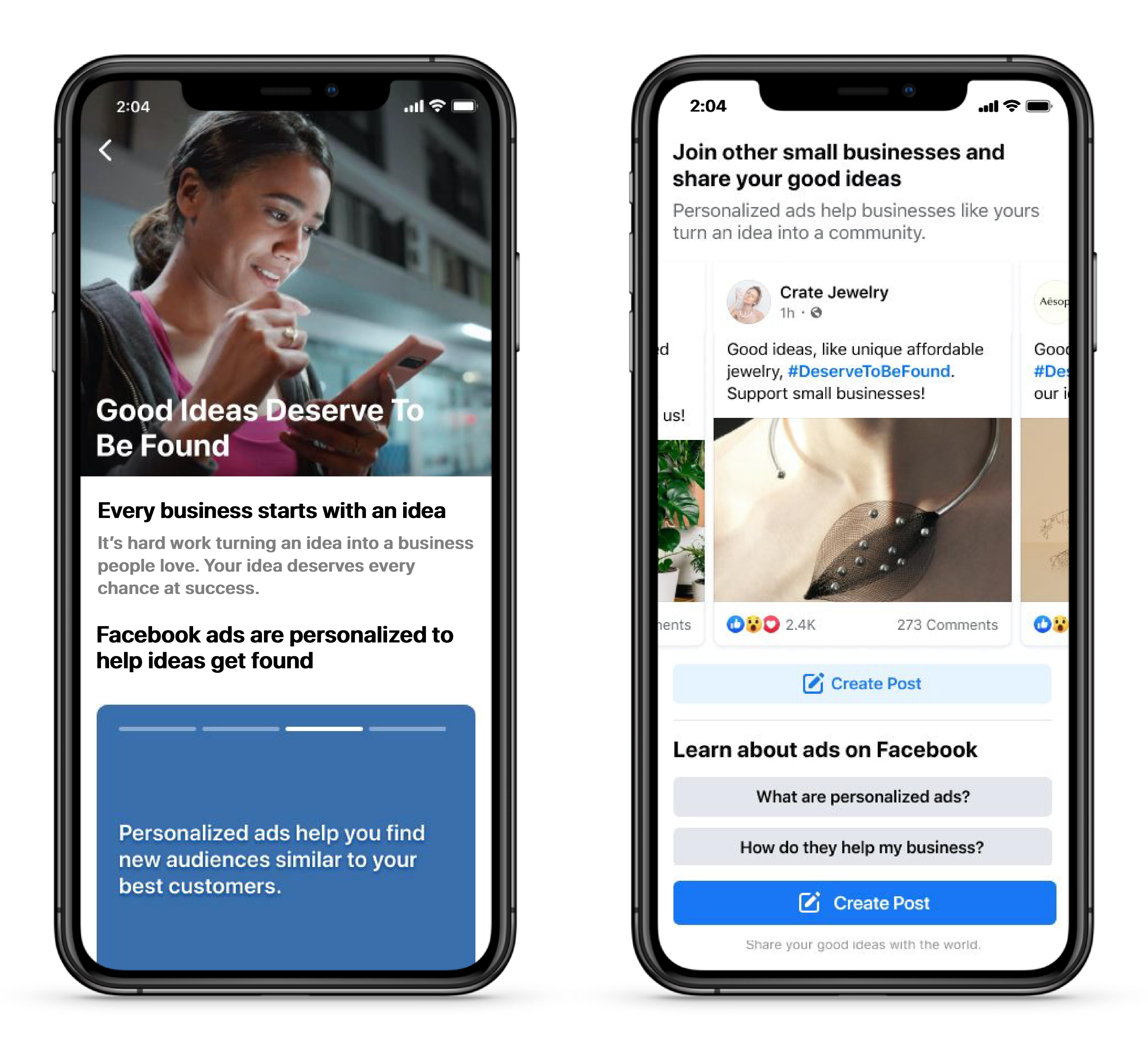The image features two iPhones placed side by side with a small gap between them. The phone on the left showcases a woman from the waist up, occupying the central portion of the screen. The image is adorned with typical iPhone interface elements: at the top left, the time reads "2:04," while the top right displays icons for battery health, cell signal strength, and Wi-Fi connectivity. An arrow pointing to the left is also visible just beneath the top icons.

The woman in the image is looking at her cell phone with a smile on her face. Her hair is pulled back into a ponytail and she is wearing a pink shirt paired with a black cardigan or hooded sweatshirt. Centered beneath her image is the slogan "Good ideas deserve to be found." 

The lower part of the phone's screen transitions to a white background, accompanied by the text: "Every business starts with an idea. Facebook ads are personalized to help ideas get found." Below this text, there is a blue button that states: "Personalized ads help you find new audiences similar to your best customers."

On the right-side phone, the screen displays a white background with the text: "Join other small businesses and share your good ideas." The bottom part of this screen features images of three different businesses, although the left and right images are partially cropped. At the center is an image captioned "Create Jewelry," alongside the text "Good ideas like unique & affordable jewelry," and the hashtag "#DeserveToBeFound." Further text encourages supporting local or small businesses with a graphic showing pieces of jewelry.

Finally, the right phone screen concludes with options such as "Create Posts," "Learn About Ads on Facebook," "What are Personalized Ads?" and "How Do They Help My Business." The bottom-most part of the screen also includes a "Create Post" button.